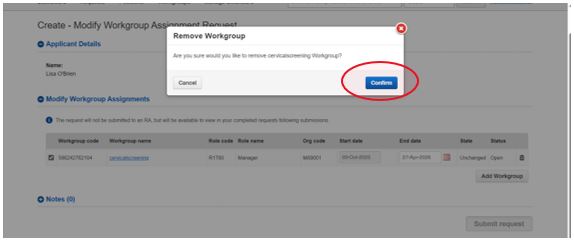In this image, we see a blurred partial capture of a website interface featuring an overlay. The background is light gray, acting as a backdrop for the main content. At the top, there's an overlay panel titled "Create-Modify Workgroup," partially obscuring the word "assignment" and possibly "work request."

The section below is titled "Applicant Details," highlighted in blue font accompanied by a blue circle. Below this, the text "Modify Workgroup Assignments" is displayed, also with a blue circle, followed by an indented blue circle indicating a sub-section or related option.

Further down, there's a gray banner with illegible information, but the terms "Start Date" and "End Date" can be discerned. Following this section is an area designated for notes, marked with a blue dot next to it. At the bottom right-hand corner of the image, there is a "Submit Request" button.

Prominently displayed is an overlaid rectangle box labeled "Workgroup." In the top right corner of this box is a red circle with an "X" inside, suggesting a close or delete function. In the top left corner, there is a "Cancel" button, while the bottom part features a blue "Confirm" button, which is circled in red pen to draw attention.